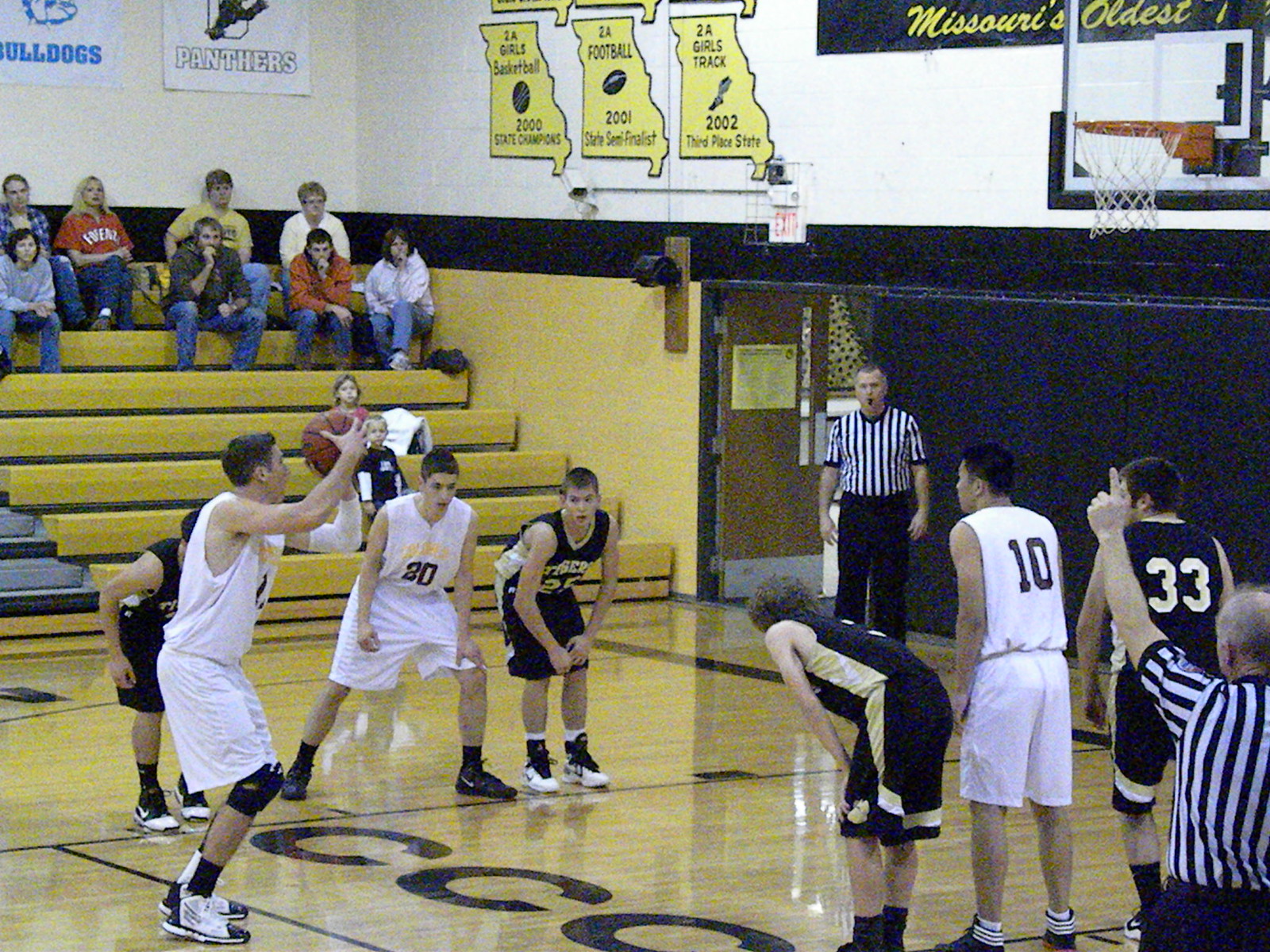In this detailed image captured during a high school basketball game in a gymnasium with yellow seats and benches, we see a player from the team in white uniforms with black lettering preparing to take a free throw with his left hand. He is leaning forward on the left side of the frame, clad in knee guards and white sneakers. Players from both teams, including those in black and gold jerseys with gold lettering, are lined up along the free throw lane, ready to box each other out for a potential rebound. The referees, identifiable by their striped black shirts and black pants, are also visible—one with a whistle in his mouth and another positioned behind some of the players. Spectators, including several women seated at the back and others sitting on the stairs, observe the game in this rather small gymnasium. Overhead, signs prominently display team names such as "Missouri's oldest Bulldogs" and "Panthers," adding a local flavor to the scene.